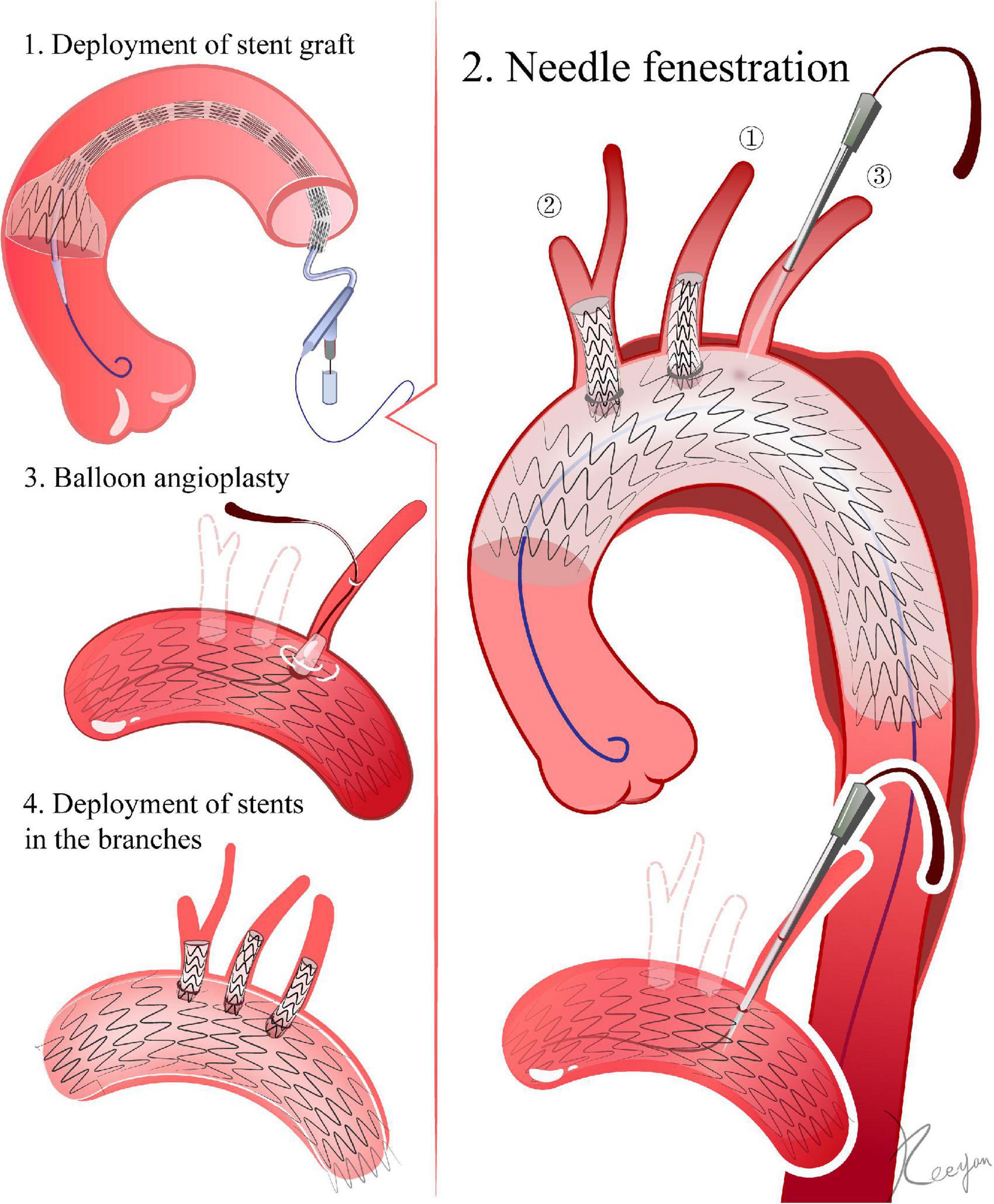This detailed medical diagram appears to be from a medical textbook and depicts a step-by-step procedure for the placement of a stent graft within a blood vessel, possibly an artery or a chamber of the heart. The diagram is hand-drawn and contains four distinct steps annotated with black text. 

1. **Deployment of Stent Graft:** In the first image, a curved, reddish-pink vessel—indicative of a blood vessel—is shown with a stent graft being introduced. A needle and a tube are depicted as they slide through the vessel, illustrating the initial phase of stent graft deployment.

2. **Needle Fenestration:** The second image focuses on needle fenestration. The vessel, again curved and pink, is now shown with various branches extending out of it. A needle and tube are once more involved, with the needle creating fenestrations (small openings) within the vessel.

3. **Balloon Angioplasty:** The third image illustrates balloon angioplasty. A structure that resembles a cross between a hot dog and a bean is shown, curved with a thin wire passing through it. This step highlights the process of widening the vessel through balloon inflation.

4. **Deployment of Stents in the Branches:** The final image depicts the deployment of stents within the branches of the vessel. It showcases a wiry, swirly object inside the branches that appears to be the stents being placed properly in their designated positions.

Overall, this detailed and sequential representation provides clear instructions on the various stages of placing a stent graft within a vascular system, showcasing the tools and steps involved from deployment through angioplasty to final stent placement in the vessel branches.